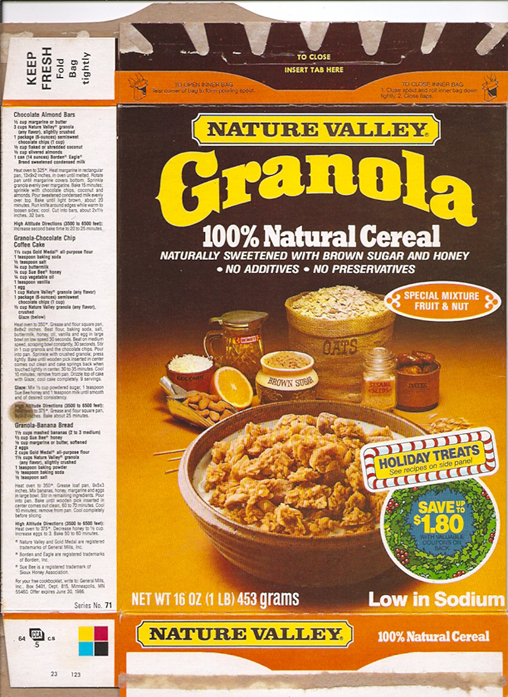In this flattened cereal box image of a Nature Valley granola cereal, the front is dominated by a yellow banner with "Nature Valley" in bold brown letters. Below it, "granola" is written in large yellow letters, followed by "100% natural cereal" in white text. The cereal is described as "naturally sweetened with brown sugar and honey. No additives, no preservatives," also in white text. The background features a vibrant image showcasing the granola in a brown bowl, surrounded by ingredients such as oats, honey in a jar, brown sugar in another jar, a sliced lemon, and potentially some almonds or peanuts. A white banner framed in red lines reads "Holiday Treats" in yellow text with blue letters, and an adjacent green and red circle promises savings of up to $1.80. Below the savings message, it states "low in sodium." The net weight of the cereal is indicated as 16 ounces or 453 grams in white text. The top edge has instructions in orange text on a yellow background that says, "To close insert tab here." The box has noticeable tear marks with patches of white, orange, and brown.